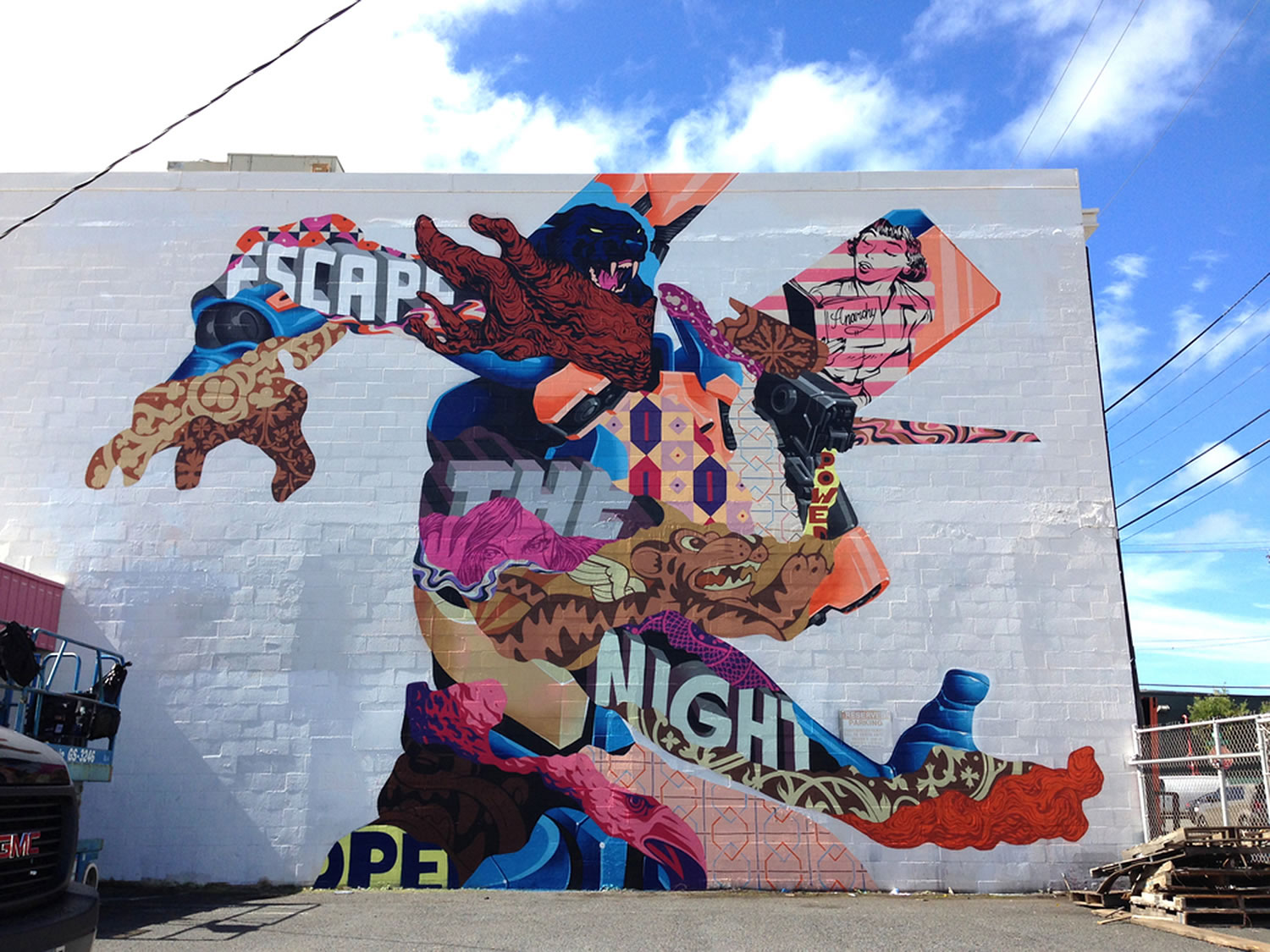In this outdoor scene, the image predominantly features a detailed mural painted on a white brick building, occupying about 80% of the frame. The upper part of the image showcases a gradient sky, transitioning from blue on the right to cloudy on the left, intersected by various electrical wires. 

The mural presents a vibrant and intricate artwork with a central theme of escape, embodied by a colossal, stylized creature that resembles a monstrous superhero. At the top left, there's the head of a black jaguar or panther, partially surrounded by what appears to be a hand. Below the head, a brown scarf extends towards the left center, with white letters spelling out "escape." The creature's left arm, painted in shades of orange, blue, and brown, stretches out from the center, holding what looks like a black movie camera.

Further down, the right arm extends to the lower right corner, exhibiting a mix of colors from red to blue, ending in a gnarled rust-colored hand with a cone-shaped thumb. The lower portion of the mural includes purple scarf-like elements wrapping around the creature’s body. 

In the middle of the mural, the word "the" is prominently displayed, while "night" is written along the right arm. Surrounding the mural are everyday urban details: a chain-link fence and metallic railings in the lower right, a GMC truck grill peeking in from the lower left, and wooden pallets. The entire scene is framed under the expanse of the sky, capturing the essence of a creatively transformed urban landscape.